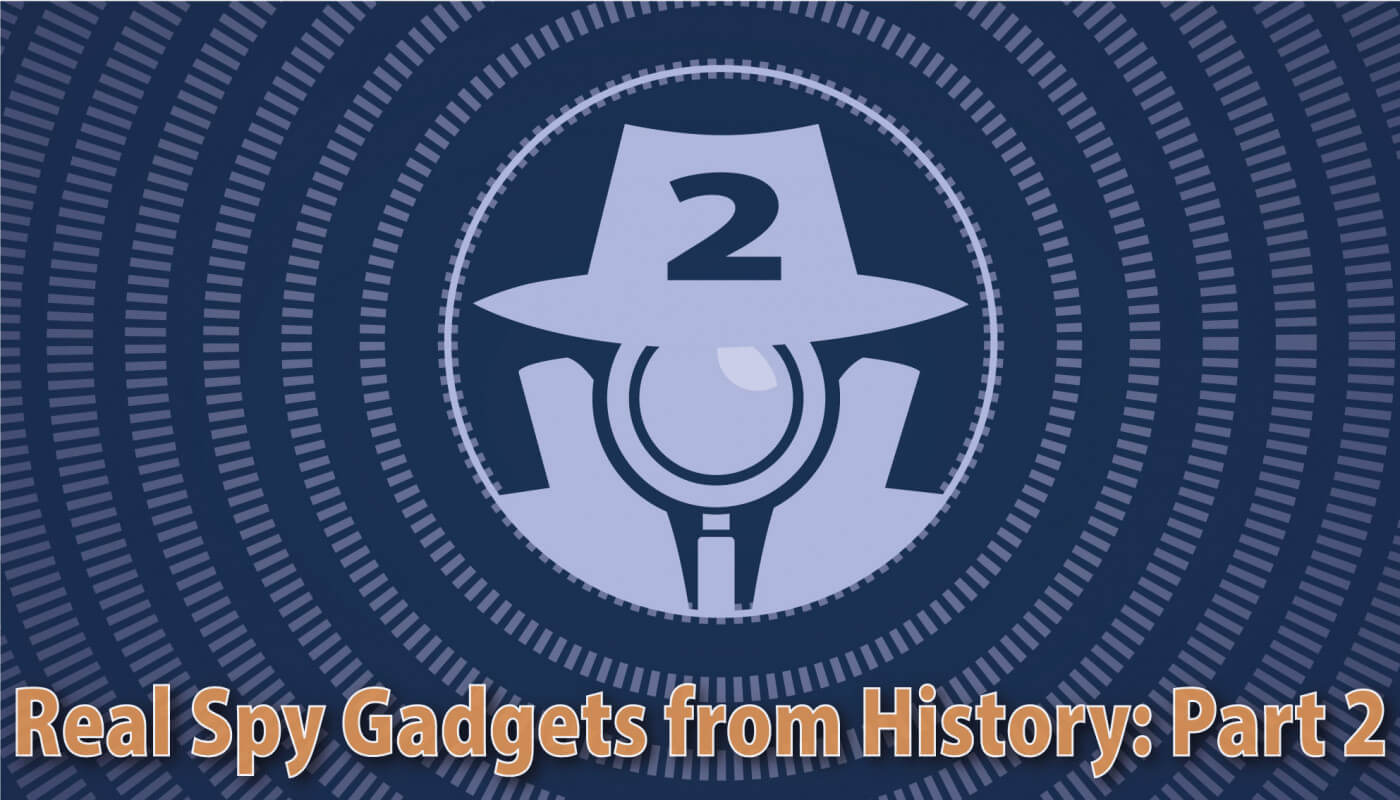The image displays a silhouette of a detective with distinct, detailed features against a predominantly dark blue or black background. The detective figure, rendered in white, wears a traditional brown detective hat marked with the number "2." Instead of a face, the head is depicted as a magnifying glass, a significant element of the design. Surrounding the magnifying glass is a collared jacket, enhancing the detective theme. The backdrop features concentric circles, creating a visual effect that resembles zooming in, with seven rings encircling the central figure. White light sun rays emanate from behind the detective, providing a radiant contrast against the dark backdrop. At the bottom, the text "Real Spy Gadgets from History: Part 2" is prominently displayed in orange, suggesting this might be an advertisement or poster for a series possibly related to spy gadgets, a game, or a TV commercial.